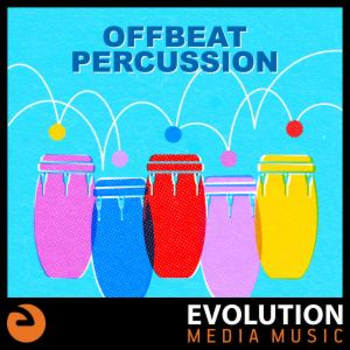This advertisement sign features a narrow black frame enclosing a light blue background. Prominently displayed at the top center in blue lettering is the text "Off Beat Percussion." Below this text is a vivid illustration of five bongos, arranged from left to right in purple, blue, red, light pink, and yellow. Each bongo has balls of matching colors—yellow, pink, blue, purple, and red—bouncing off their surfaces, connected by white arches and lines, suggesting motion. At the very bottom, there is a narrow black band. On the left side of this band is a small red circular logo, and on the right side, the text "Evolution" appears in white, with the words "Media Music" written in red beneath it.